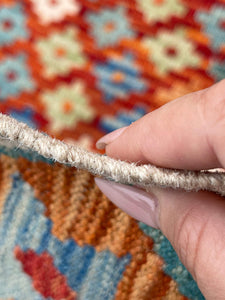In this close-up photograph, a woman with freshly manicured, light pink nails holds the edge of a meticulously crocheted rug between her thumb and pointer finger. The beige edge of the rug she is holding is highlighted against a vibrant and intricate background. The rug features an elaborate pattern composed of mainly orange and red hues, interspersed with diamond-shaped designs. These diamonds display varying colors, such as blue with orange centers and white with red centers. The diamonds are intricately sectioned by a predominant red fabric, with each diamond seemingly adorned with colorful dots. The juxtaposition of her clean, polished nails against the rich, colorful texture of the rug creates a visually striking image, emphasizing both the craftsmanship of the crocheted material and the elegance of her well-groomed hands.